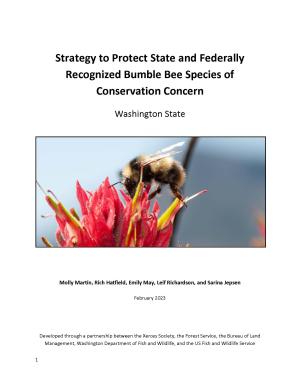The image is a detailed advertisement or pamphlet depicting a bumblebee on a flower, zoomed in and centrally placed within the rectangular frame. The bee, characterized by its yellow with black stripes and transparent wings, is perched on a bright red or pink flower. The photograph itself appears somewhat blurry, with the flower being the most focused element. The background behind the flower and bee is an extremely blurred blue-gray, possibly hinting at buildings or a skyline but not distinctly clear. Surrounding the photograph, the background of the overall image is white. Above the photograph, large, black text reads: "Strategy to Protect State and Federally Recognized Bumblebee Species of Conservation Concern, Washington State." Smaller, unreadable text can be found beneath the photo. This layout and detailed visual presentation suggest the image could be a page from a book or a conservation pamphlet.